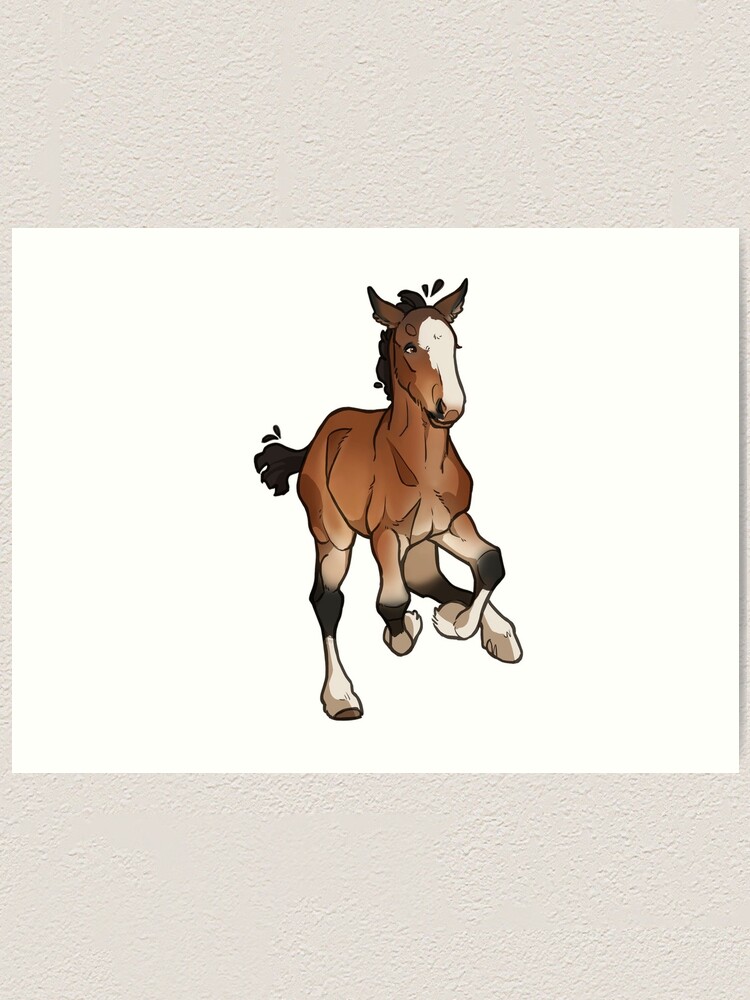The image features a color illustration of a galloping foal centered on a white piece of paper. This paper is mounted on a textured, off-white wall. The foal, depicted in a cartoon style, has a coat that transitions from dark brown to lighter shades. Its mane and tail are black, while the legs are a gradient of black to white, with shaggy fetlocks above black hooves. A distinctive white stripe runs down its nose. The foal appears focused and serious as it leaps forward, with both front legs raised. There are no additional elements such as text, people, animals, or buildings in the illustration.